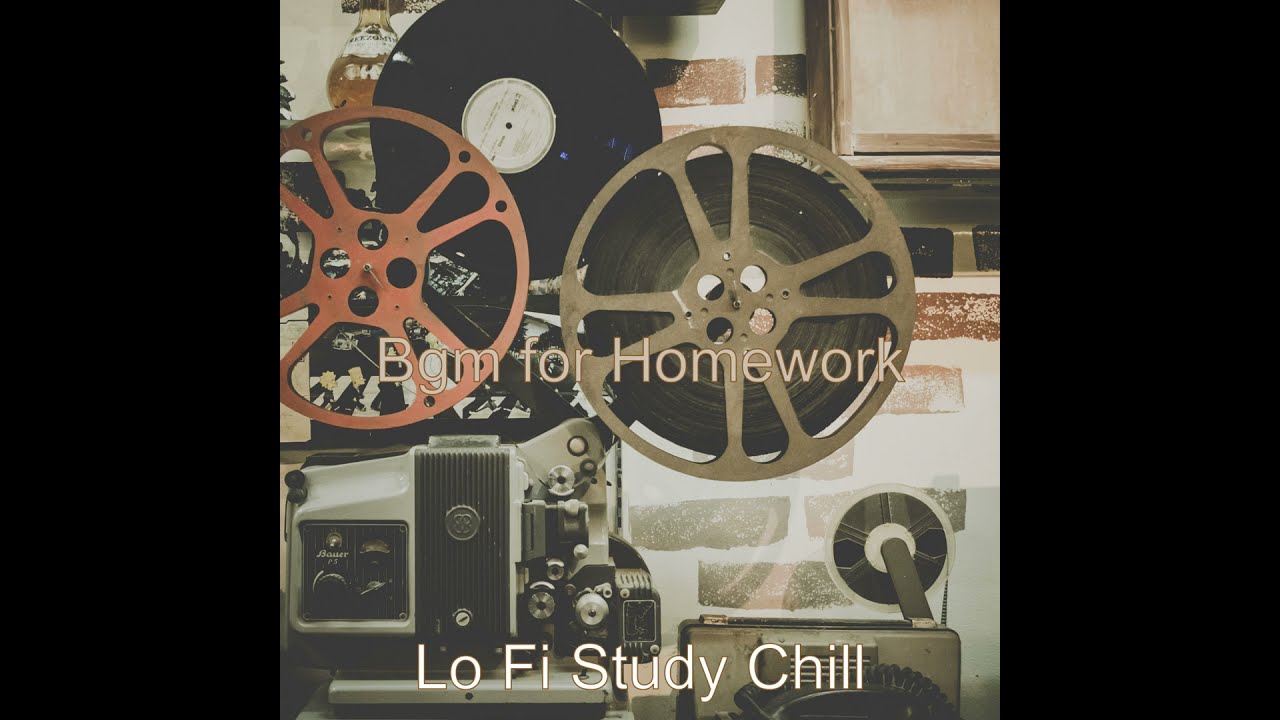In the sepia-toned image, we have a horizontally rectangular frame with black borders on either side. At the center, the focal point is an old-time movie projector, featuring prominently its two large reels, one on the left-hand side colored red and the other on the right in a dull grey. The projector, detailed with various knobs and mechanisms, sits among other electronic equipment on what appears to be a counter, possibly in a kitchen setting. A faux brick wall backdrop accompanies the scene with off-white lettering directly on it, stating "BGM for homework" with the letters 'B' and 'H' capitalized. Below this, in white block letters, the text reads "lo-fi study chill," with each word starting with a capital letter. The image gives off a vintage vibe, entirely presented in different shades of sepia, highlighting the nostalgic feel of an old newsreel or vintage media setup.